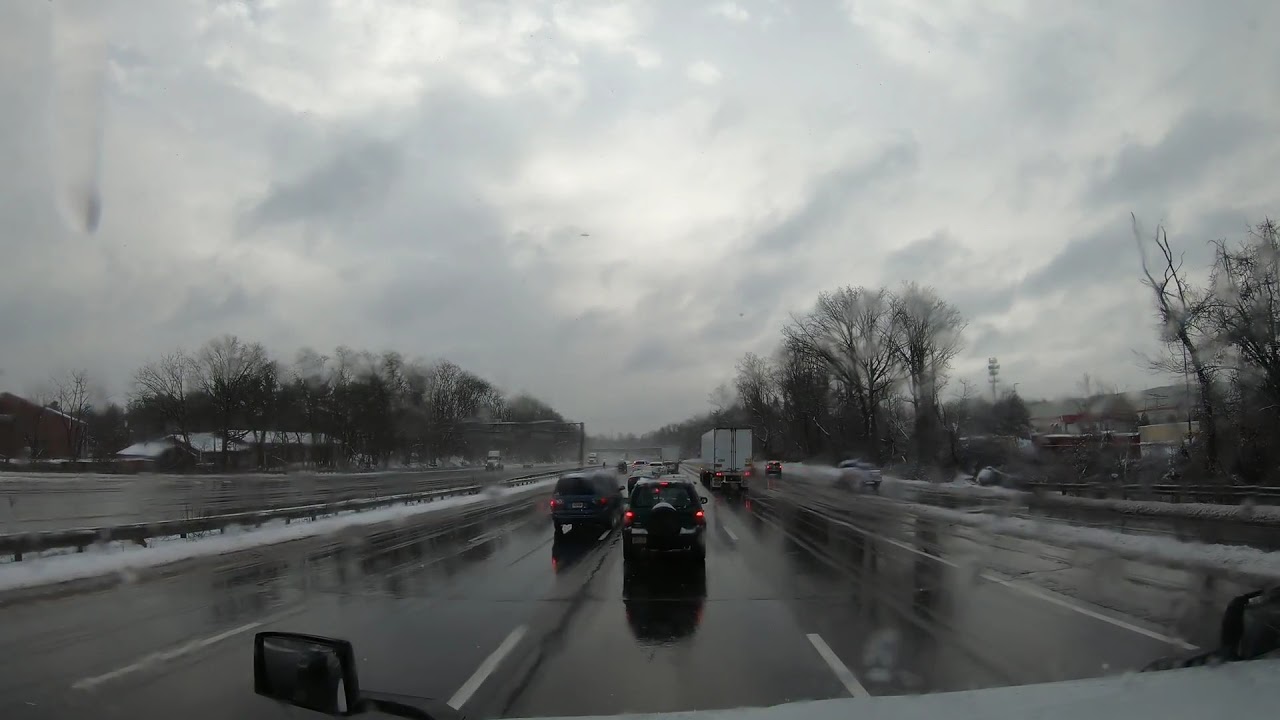This image, likely captured from the vantage point of a car's dashboard camera, offers a wide and detailed view of a multi-lane road on a rainy winter day. The perspective shows the road ahead receding towards the horizon line just under the middle of the frame, flanked by a black metal object visible at the bottom left and right corners, presumably parts of the car. The road, glistening with puddles and reflecting the gray sky above, is segmented by white lane markings. Snow is scattered along various parts of the road and cars ahead, adding to the wintry atmosphere.

To the left, a parallel several-lane road runs in the opposite direction, relatively clear of traffic, in contrast to the lanes in view which are backed up with vehicles, possibly due to a stoplight, traffic congestion, or an accident. The sky is predominantly overcast with clouds, though patches of light blue are visible. Ahead, two SUVs are directly in front, with a white transport truck and additional cars visible in the traffic. The standings trees lining the road are bare, indicating dormant winter state, and a few distant businesses can be faintly seen in the background. This comprehensive view captures both the stillness of traffic and the subtle movement in the landscape, presenting a stark, yet detailed portrayal of a winter's day on the road.